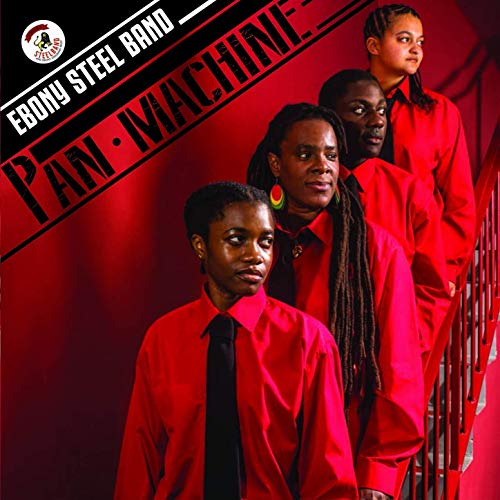The image depicts an album cover titled "Pan Machine" by the Ebony Steel Band. The design mimics the iconic album by the German band Kraftwerk, "Man Machine," but presents a tropical twist. In the top left corner, the title "Ebony Steel Band" is written diagonally in white text on a black background, beneath which the album name "Pan Machine" is displayed in black text on a red background. The cover features four Black women standing on a red staircase with metallic steps at the bottom and a red railing. They are dressed in red business suits with black ties, and most have braided or dreadlocked hair. Notably, one member, who is the second to last from the top, wears large, round earrings in vibrant orange, yellow, and green colors. All four women gaze to the right, bringing a cohesive and striking visual to the album cover. The woman at the top has the lightest skin tone among the group. The background behind them is entirely red, emphasizing the tropical reimagining of the Kraftwerk homage.